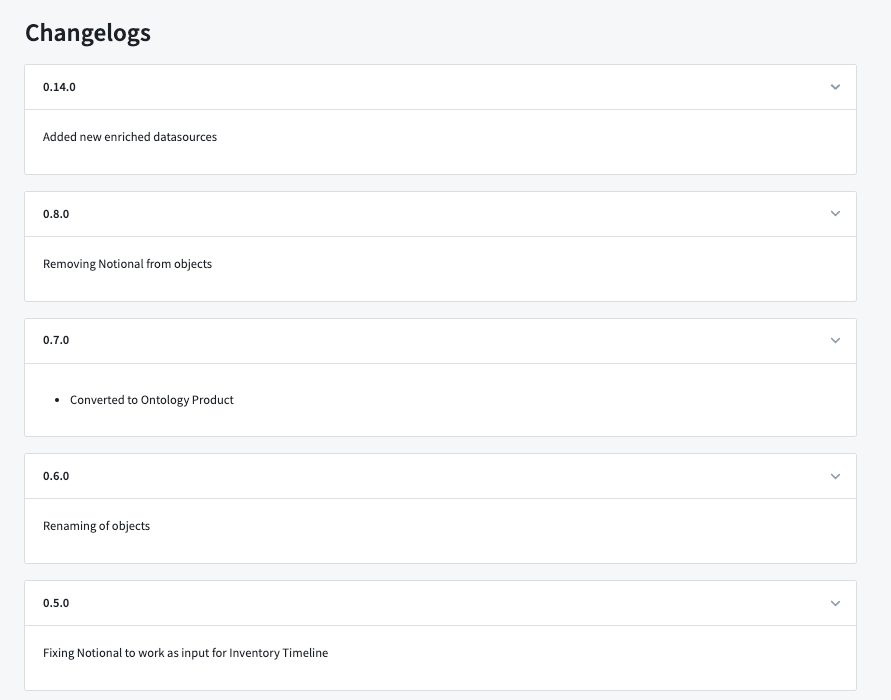"Screenshot of a change log document with a light off-white background and a hint of gray. The document is structured into multiple sections, each detailing version updates:

- At the top, the title 'Change Logs' is displayed clearly. 
- The first section features '0.14.0' in bold black on the left side, accompanied by a downward-pointing arrow to the right. A thin line spans horizontally under this heading.
  - Beneath, it lists 'Added new and enriched data sources.'
  
- The next section begins with '0.80' in bold black on the left, again with a downward-pointing arrow on the right, and a thin gray line underneath.
  - It notes 'Removing notional from objects.'
  
- Following this, '0.70' appears in bold black on the left, with a downward-pointing arrow to the right.
  - This section mentions 'Converted to ontology product' next to a bullet point.
  
- Further below, '0.60' is displayed on the left with a downward-pointing arrow to the right and a separating line dividing it from the previous section.
  - This part states 'Renaming of objects' in black text.
  
- At the bottom, '0.50' is indicated on the left with a downward-pointing arrow on the right, followed by a thin line. 
  - It specifies 'Fixing notional to work as input for inventory timeline.'